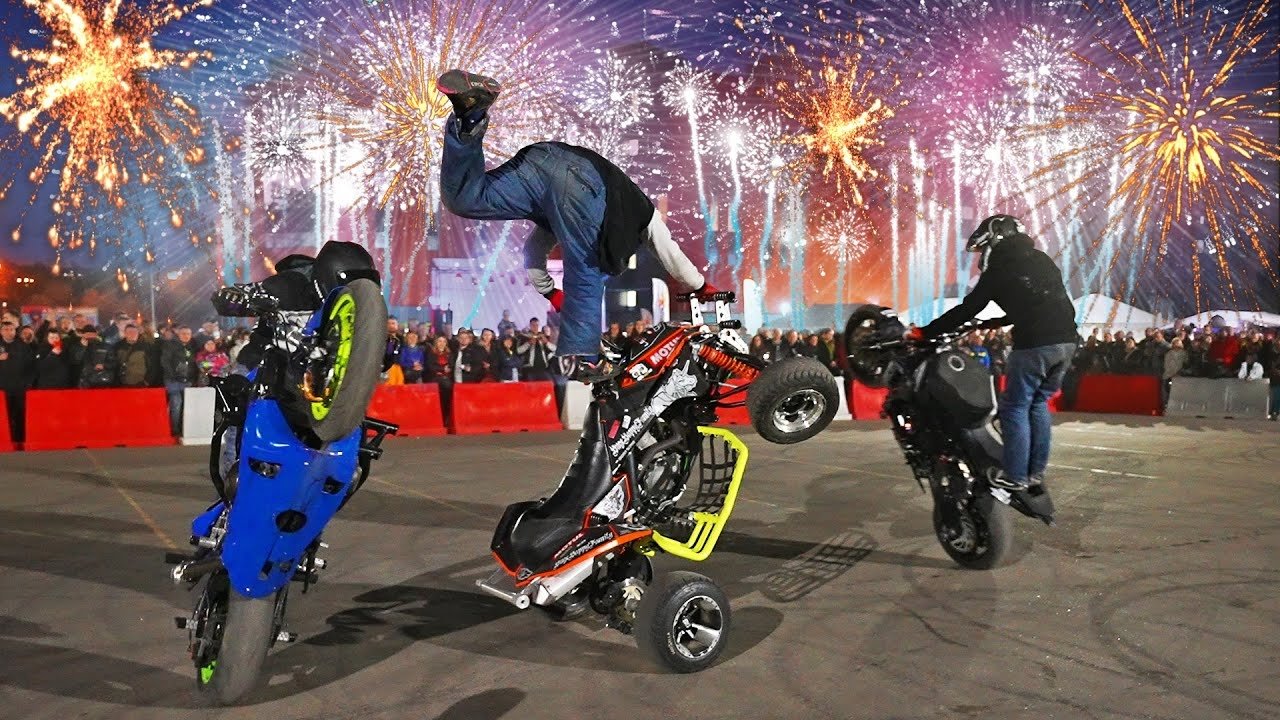This is a vibrant color photograph of a thrilling outdoor motorcycle stunt performance at a large public venue. Three bikers, donning black jackets and helmets, are executing gravity-defying tricks on their bikes amidst a crowd. On the left, a rider on a blue and black motorcycle is popping a wheelie, his right elbow barely visible as he balances the bike. In the center, another performer on a red, black, and yellow four-wheeler is standing impressively on the handlebars, his left foot elevated dramatically. The biker on the right, riding a black motorcycle, is executing a wheelie while standing on the seat, facing away from the camera. The scene is set against a backdrop of an expansive orange building and several white and gray tents. Red and white barricades separate the performers from the large, enthusiastic crowd, many of whom are capturing the moment on their iPhones. Overhead, a dazzling display of white and gold fireworks illuminates the blue sky, adding to the electrifying atmosphere.